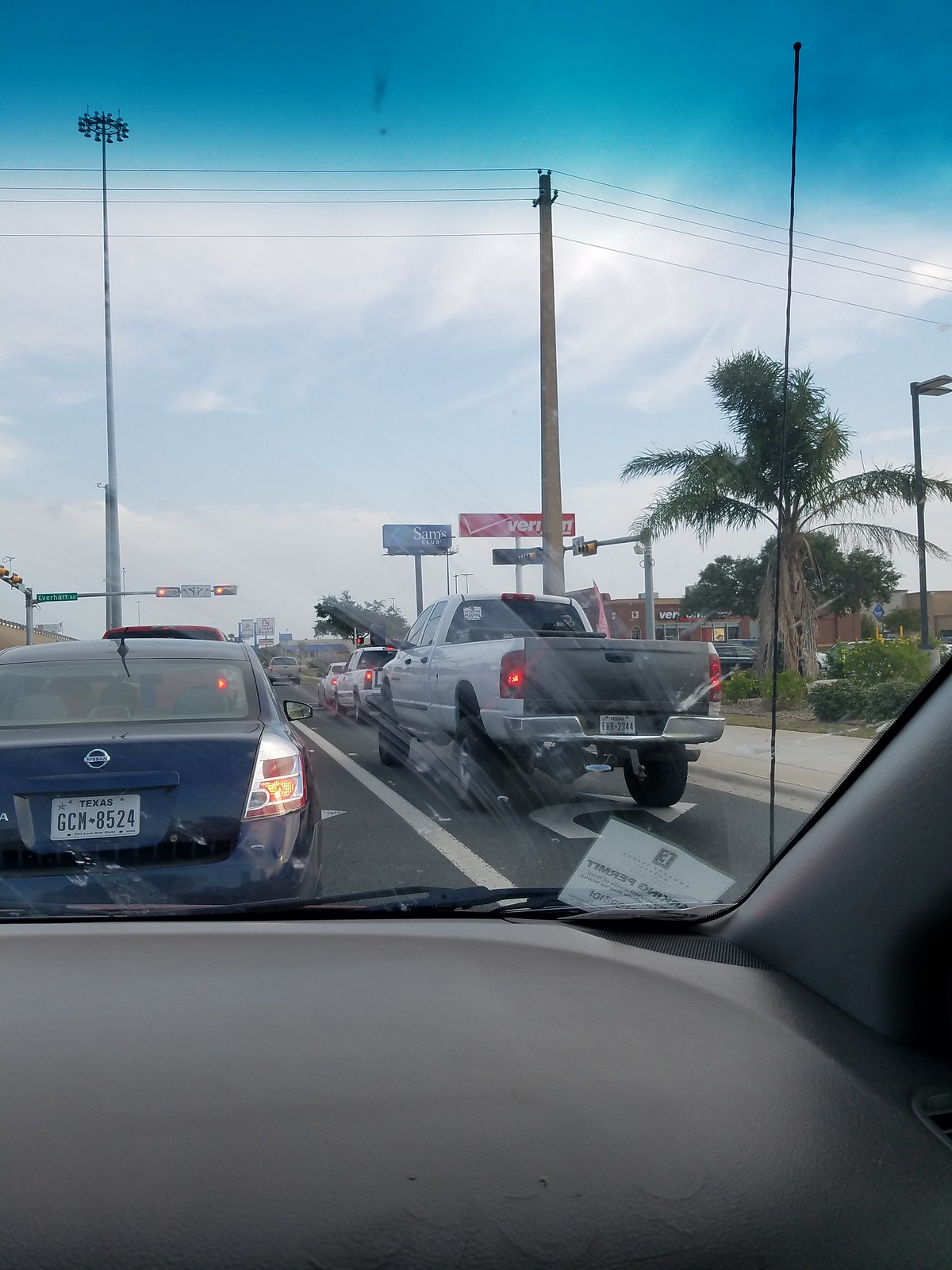This color photograph, captured in portrait format from the front passenger seat of a vehicle, offers a detailed view of a traffic-laden street scene. Taken through the windshield, the image prominently features a blue Nissan with the Texas license plate GCM 8574 directly ahead. In the adjacent right lane sits a large, silver pickup truck with a bed that has a mismatched black door. Both vehicles, along with others further ahead, are stopped at a red light. On the far right, a substantial concrete pole extends lines above the traffic, while a palm tree is visible further along the roadside. The landscape is dotted with various billboards, including a prominent red Verizon Wireless sign and a blue Sam's Club sign, reflecting a commercial, albeit unattractive, area. The dashboard of the capturing vehicle, seen at the bottom of the image, appears gray with a partially visible white sticker bearing black lettering, which is indistinct. The sky above is a vibrant blue with scattered clouds, adding a touch of brightness to the urban setting.